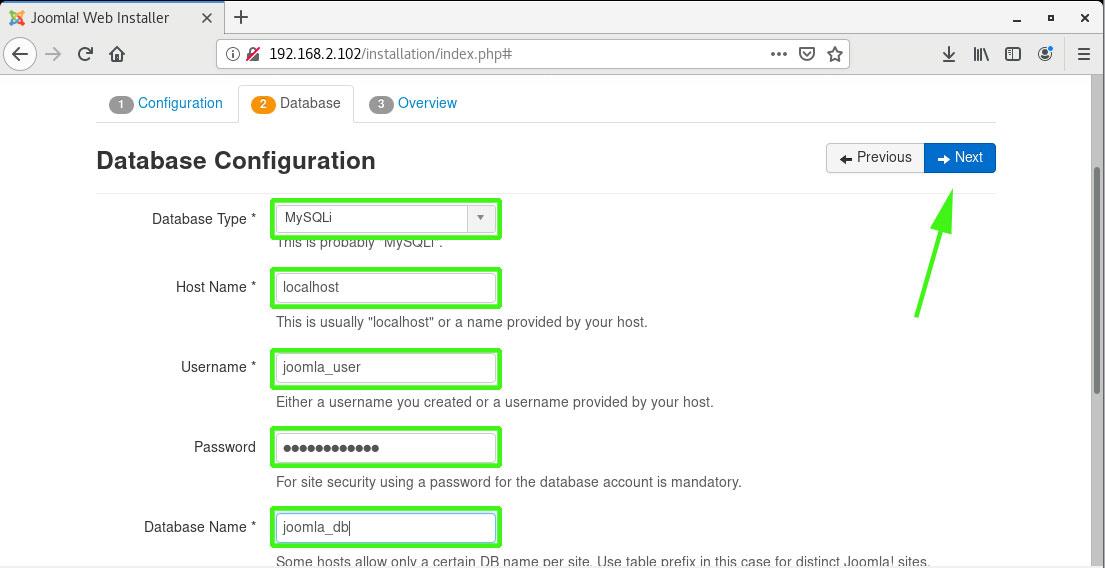At the very top left of the image, there is an 'X' symbol with its lines positioned from the top-left to bottom-right in red, and another from the bottom-left to top-right. The text "Joomla Web Installer" is prominently displayed along with another 'X' and a plus sign. On the right side, there are icons for minimize, maximize, and close.

To the left, navigation arrows (left and right) are visible, followed by a 'swoop' icon, a house icon, an eye icon, a dark gray lock with a red slash through it, and a URL: "192.68.2.102/installation/index.php#". A gray circle with an ellipsis, a shield with a checkmark, a star, a down arrow, a line, and icons resembling books are also part of the scene.

The main content area shows sections titled "Configuration," "Database," "Overview," and "Database Configuration." Within this, there is a rectangular area with navigation buttons labeled "Previous" on the left and "Next" on the right, which is highlighted in blue. 

The "Database Type" field is highlighted in green, indicating "MySQLi," typically referring to MySQL Improved. Other database details include:
- Hostname: "localhost"
- Username: "Joomla user"
- Password: obscured by dots for security (e.g., "123456" represented as ••••••)
- Database name: "Joomla_db"

There are also icons of left and right arrows with a green arrow pointing to the blue rectangle containing the "Next" text, indicating a progression step in the installation process.